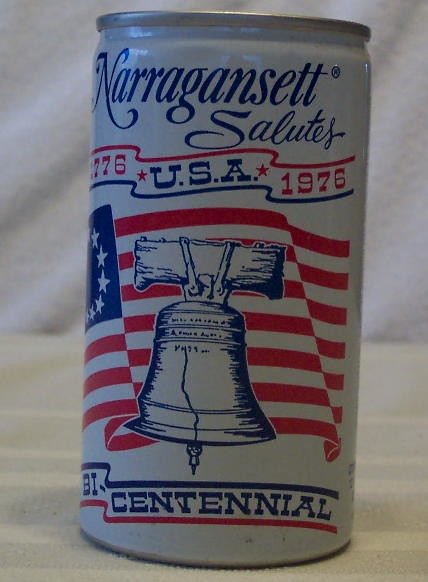The image showcases a white can with blue and red writing, prominently featuring patriotic themes. The can, which is a cylindrical shape, is positioned on a light brown wooden table against a white background. At the top of the can, in blue text, it reads "Narragansett Salutes" with a small circle R above "Narragansett". Beneath this, a banner with the inscription "1776 U.S.A. 1976" spans the can, with the years written in red and "U.S.A." in blue. Central to the design is an American flag, which has horizontal red and white stripes and a blue square with white circular stars. Superimposed over the flag is a blue and white Liberty Bell. Below this imagery, the word "Bicentennial" is written in blue, flanked by wavy red and blue lines. The can rests on a table, and a white sheet is draped in the background, giving the scene a clean, focused aesthetic.